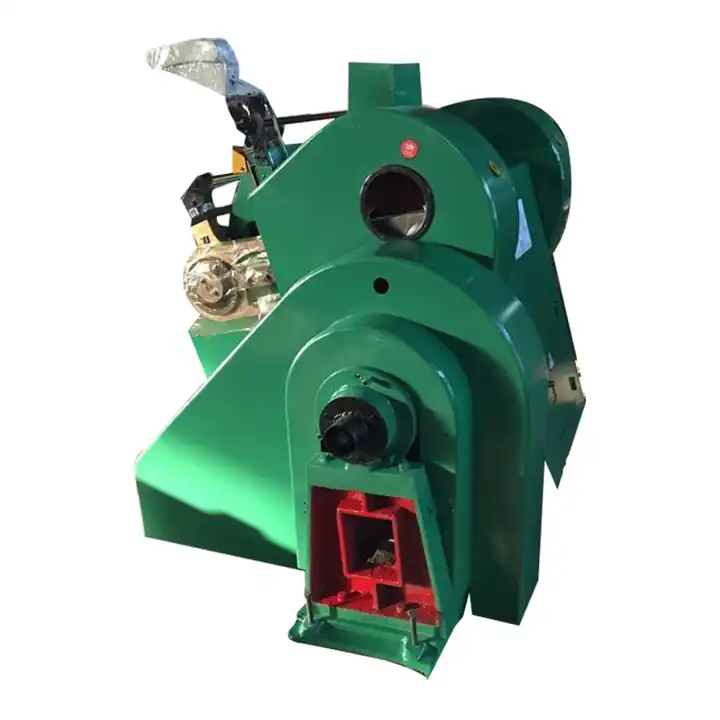This image portrays a close-up of an industrial device that appears to be a component of a larger machine, possibly a winch or electric motor drive. Predominantly green in color with both light and dark green sections, the device features a noticeable red area at the bottom. This red section includes an indented, squarish opening that seems designed for fitting or attachment. Above this, a round black nut, likely a screw-in component, can be seen. The machine's intricate structure includes a black shaft in the center and another small black opening above it. On the back left, there are silver metal pieces extending, resembling blades but likely non-functional in that capacity. The bottom left portion of the device catches sunlight, giving it a lighter green appearance. The entire apparatus, made from tough, heavy metal, suggests robust industrial use and could weigh about half a ton. The background shows a white filter effect, indicating sunlight interacting with the machine.